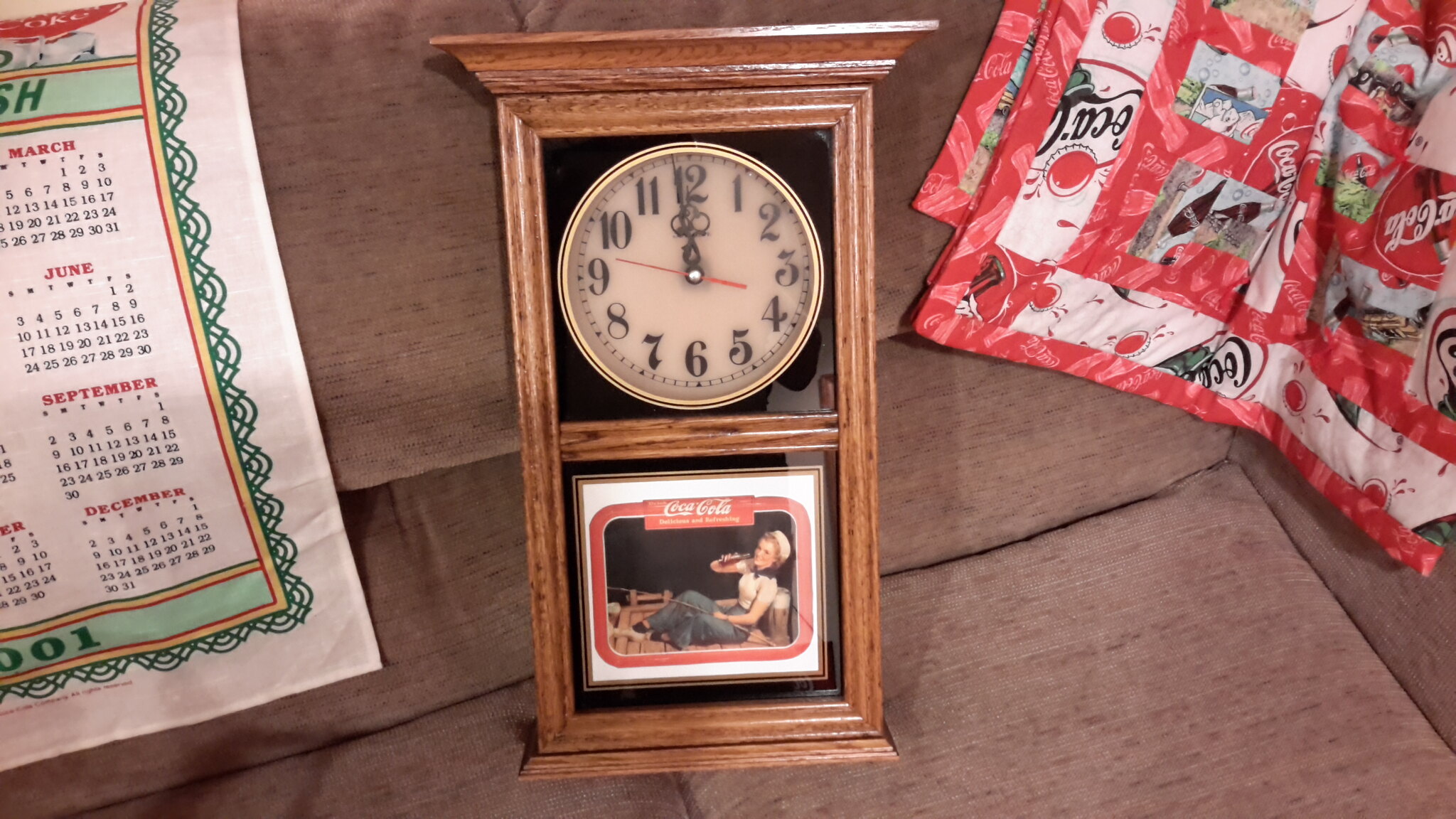In the center of this indoor photograph, a small, ornate wooden desktop clock is prominently displayed on a worn, brown fabric couch with intricate lines and shades giving it a dimensional appearance. The clock, shaped like a rectangle, features an off-white face with black serif numbers and elegant black metal hands with three circular rings, as well as a red second hand. The clock reads 11:59. Below the clock face, the clock's wooden frame showcases a vintage Coca-Cola advertisement of a woman dressed in a naval outfit—complete with a hat, white shirt, and denim pants—cheerfully drinking from a Coca-Cola bottle, with just the paws of her dog visible at her feet. The advertisement includes the iconic Coca-Cola logo in white on a red, rounded rectangle. To the left of the clock, draped over the couch, is a white cloth calendar adorned with ornate green swirls and displaying the months of the year. On the right side of the clock, a red, white, and black Coca-Cola quilt or blanket featuring various images of Coca-Cola products is casually flung over the couch.